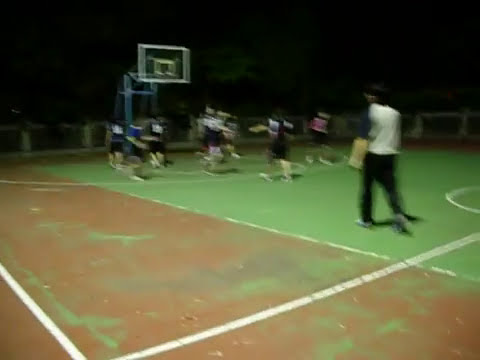The photograph is a very blurry, nighttime image of a kids' basketball practice on an outdoor cement court. The scene captures a group of young players, some in black jerseys and others in different colored shirts, gathered around a solitary basketball hoop positioned towards the left side. The unfocused background is predominantly black, hinting at the late hour, with a faint outline suggesting a fence. There is also a hint of tree leaves under the dark sky. On the right side, slightly forward of the group, stands a man with dark hair, facing the kids, likely the parent coach overseeing the practice. He is dressed in a white top and black pants. The court itself appears worn, with rough patches that might benefit from repainting.